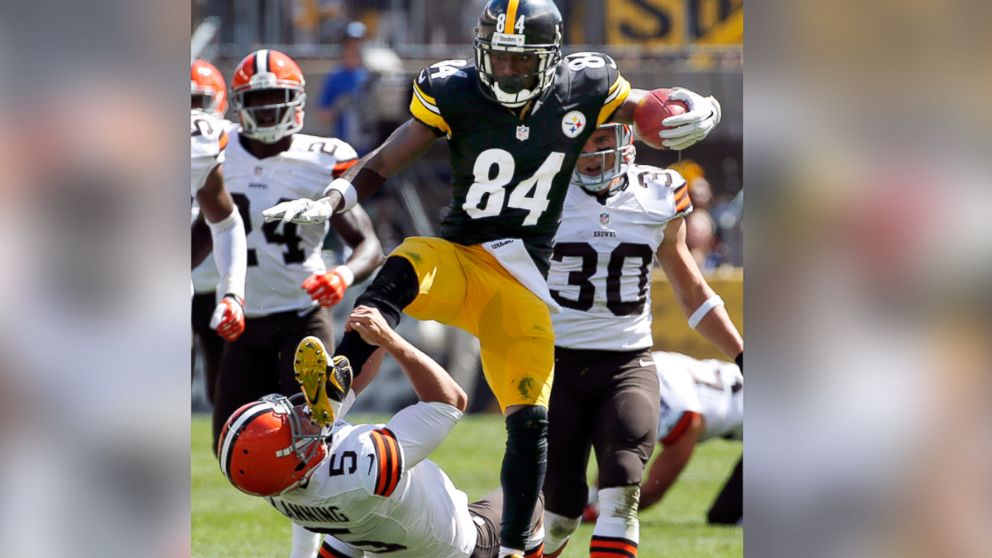The image depicts an intense moment during a daytime football game, likely featuring the Pittsburgh Steelers against the Cleveland Browns. In the center, a football player donning a black jersey and bearing the number 84 in white is captured in mid-action. He is holding a reddish-brown football securely between his left forearm and hand. This player, identifiable by his dark helmet with the same number, has one leg raised, inadvertently or intentionally striking the face mask of an opposing player who wears a white jersey and red helmet marked with the number 5. The stricken player is midway through falling backwards, having already landed on his rear with his teammates a few steps behind, rushing to the scene. The background of the image shows a grassy field, blurred spectators, and a hint of stadium infrastructure, including possibly a TV camera capturing the intense gameplay. The immediate impact and dynamic motion are crystallized by the clear focus on the central action amidst the hazy peripheries.